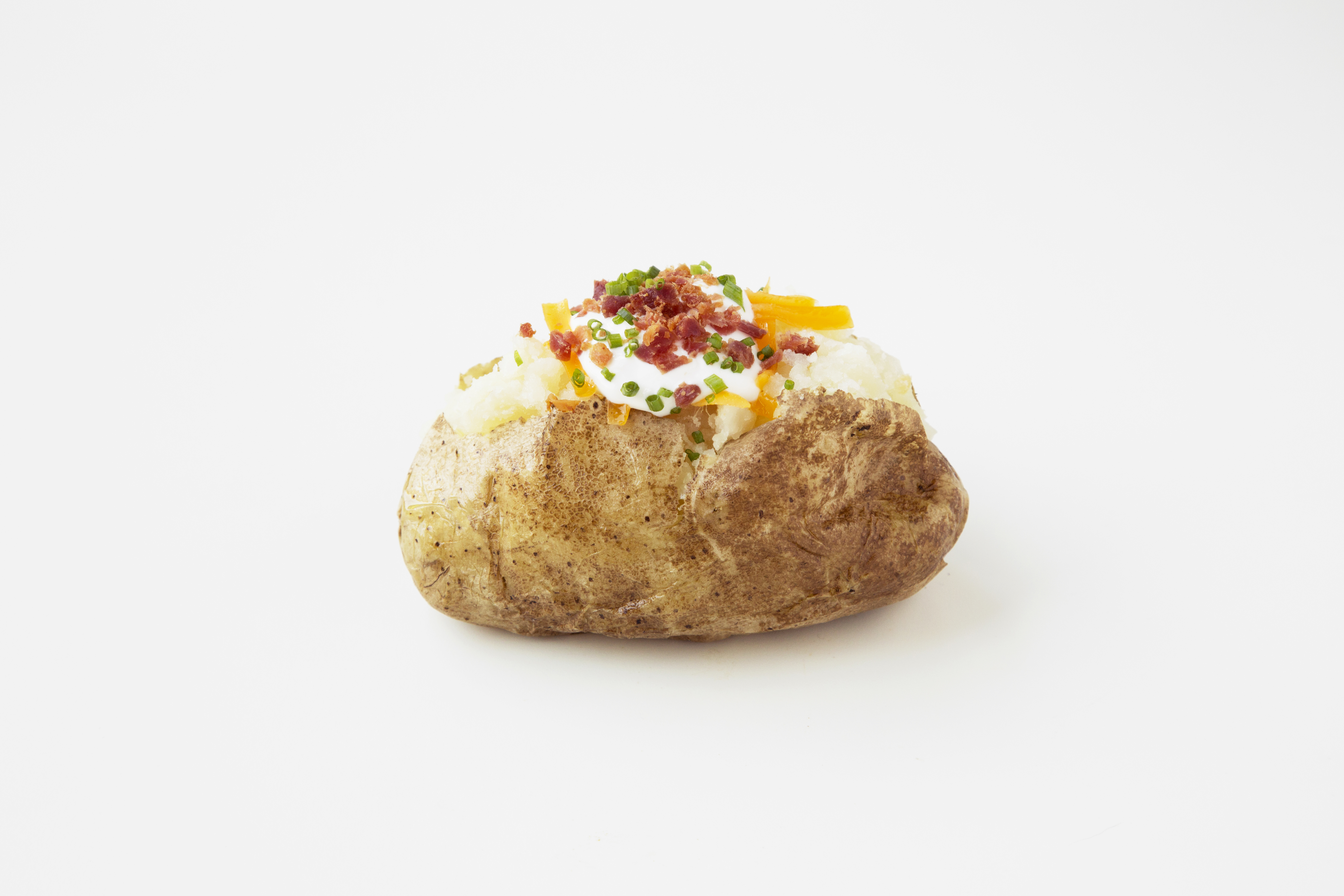The photograph showcases a medium-sized baked potato on a pure white background, centered in the frame. The skin of the potato is a baked, browned texture, indicating it may be a russet variety. The potato is split open down the middle, revealing its fluffy white interior. Piled into the center of the potato is a generous "loaded" topping of white sour cream, shredded cheddar cheese in a deep yellow-orange hue, finely chopped green chives, and bits of dark red-pink bacon. The toppings form a flavorful, colorful mound that highlights the potato's delicious innards, emphasizing the classic appeal of the loaded baked potato.